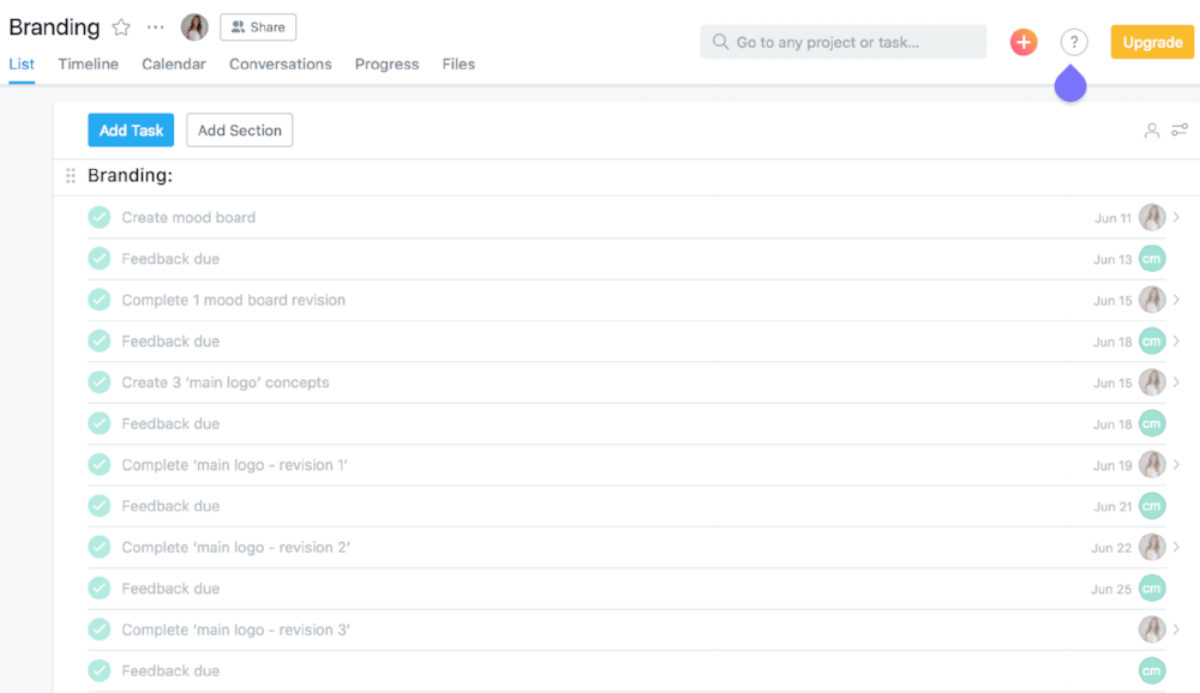On a minimalist white background, the upper left corner features the word "Branding" in bold black text. Adjacent to this, there is an empty star icon, indicating a favorite selection option, accompanied by a horizontal gray three-dot menu icon, and a miniature profile image of a woman wearing a white top. Next to these elements is a gray "Share" button inside a white box.

Below this section, there are selectable categories labeled "List," "Timeline," "Calendar," "Conversations," "Progress," and "Files," with "List" being highlighted in blue as the selected category. To the right, a blue button with white text reads "Add Task," alongside a white button with gray text reading "Add Section."

Further down, the word "Branding" appears again in bold, followed by a list of tasks: 
- "Create mood board" with a "Feedback due" label.
- "Complete one mood board revision" with a "Feedback due" label.
- "Create three main logo concepts" with a "Feedback due" label.
- "Complete main logo revision one" with a "Feedback due" label.
- "Complete main logo revision two" with a "Feedback due" label.
- "Complete main logo revision three" with a "Feedback due" label.

Each task on the right-hand side features associated profile icons.

In the upper right corner, there is a search bar reading "Go to any project or task" flanked by a plus sign. Next to it, a purple dot points to a circle containing a question mark, and a yellow "Upgrade" button is present.